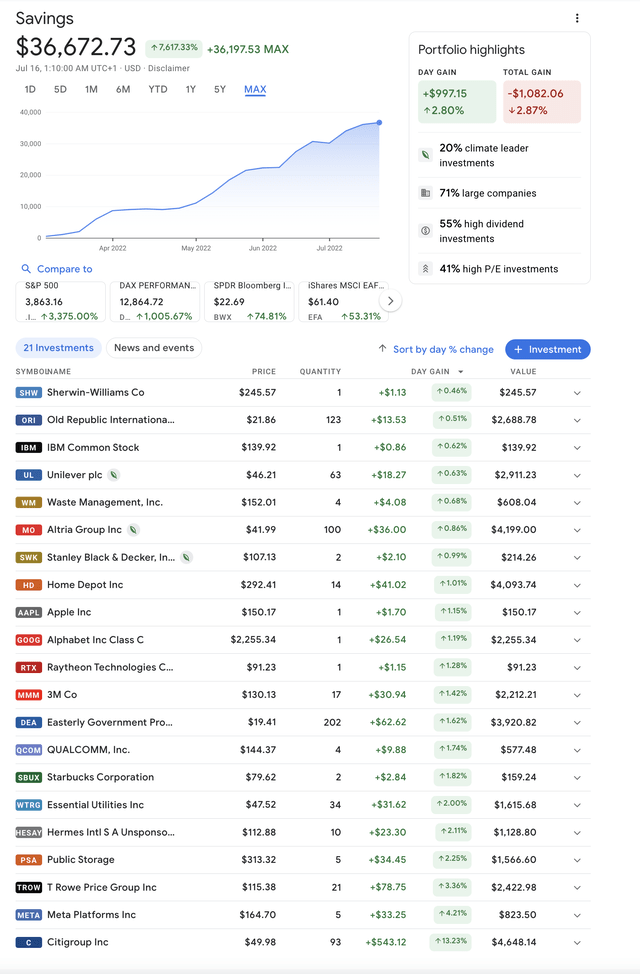This image captures a screenshot of a financial portfolio dashboard. At the top of the screen, prominently displayed, is the current portfolio value of $36,672.73. There are various sections with financial data and metrics. Toward the upper section, the dashboard shows a performance summary highlighting gains, including day gains and total gains.

The left sidebar features a "Portfolio Highlights" section, presenting investment categories such as 20% Climate Leader investments, 71% Large Companies, 55% High Dividend investments, and 41% High P/E investments. A visual line graph charts the portfolio's growth, showing a continuous upward trend from April 2022 to July 2022, peaking at approximately the $40,000 mark.

Below the graph, the dashboard lists specific stock details, including symbols, names, and related financial information. Examples include companies like Sherwin Williams, Old Republic International, and IBM Common Stock. Each listed entry provides details such as the stock price, quantity, day gains, and overall value, enhancing the comprehensiveness of the financial overview.